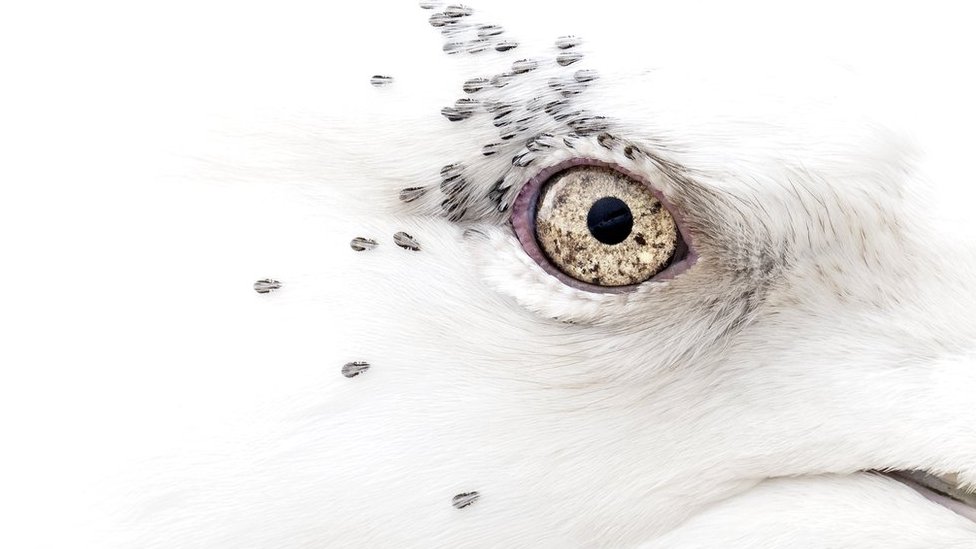The image presents an extremely close-up view of an animal's eye, most likely a canine or a bird, based on the white fur or feathers surrounding it. The eye itself is detailed and intricate, with a distinct black pupil at its center. Encircling the pupil is an iris displaying a gradient of colors, predominantly gold and yellow, interspersed with glitter-like sparkles and occasional black speckles. The eyelid is tinged with a pinkish hue, and tiny black dots are embedded in the skin around the eye, resembling small teardrop shapes. The fur, or possibly feathers, in the vicinity of the eye appears fluffy and soft, predominantly white, with occasional hints of black and gray hair. To the right of the eye, there is a gray slit, which might be part of the mouth or beak, suggesting the head of the animal extends outwards in that direction. The landscape-oriented image, characterized by its detailed and textured depiction, captures the striking and complex features of the animal's eye, making identification challenging but highlighting the beauty in its minutiae.